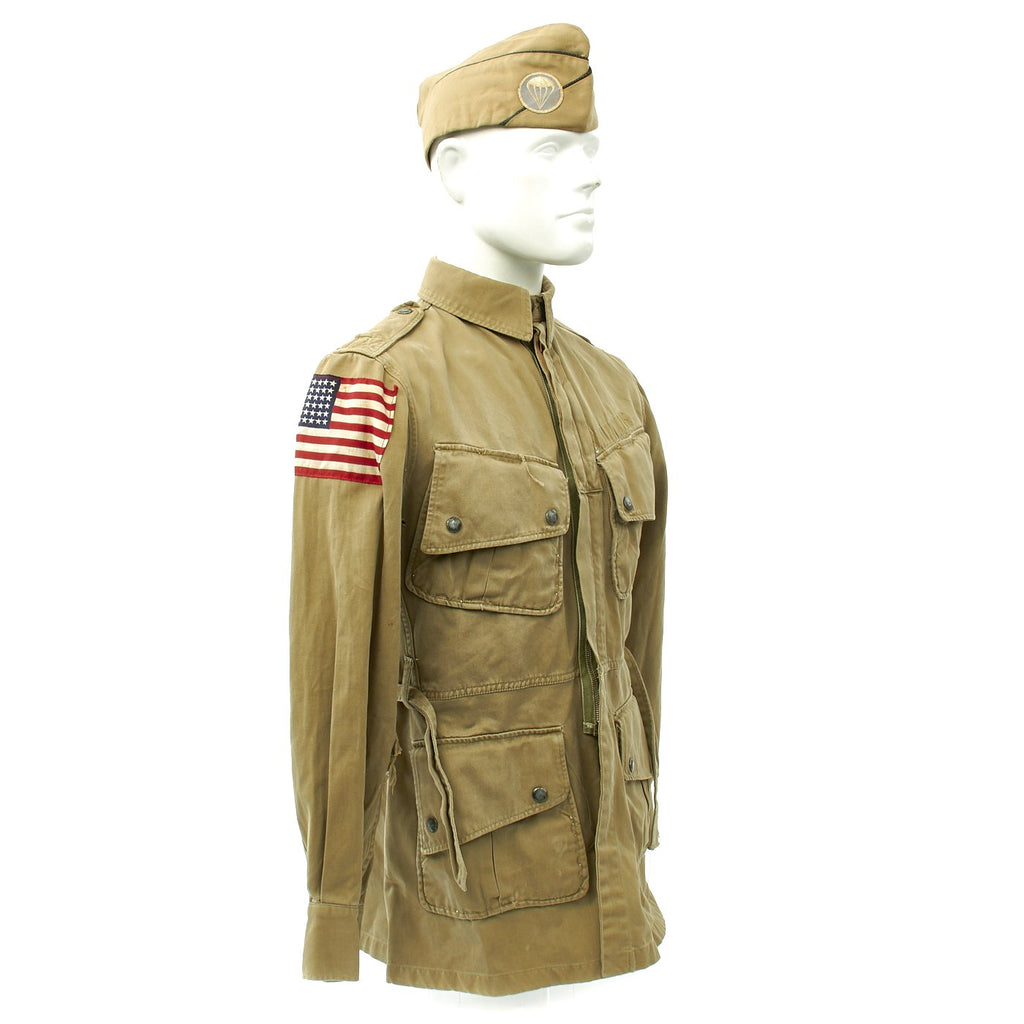This photograph captures the upper half of a stark white mannequin adorned in a military uniform. The mannequin's head is slightly tilted forward and angled to the right, featuring minimal facial details except for contours around the ears, eyes, nose, mouth, and eyebrows. It wears a light brown beret with an emblem at the front, which appears to be a yellowish circle with a parachute design. The mannequin is dressed in a khaki-colored jacket that has a casual style and is zipped all the way up to the collar. The jacket boasts multiple pockets – two on each side of the chest. Prominently displayed on the right shoulder of the jacket is a large American flag patch, adding a patriotic touch to the ensemble.